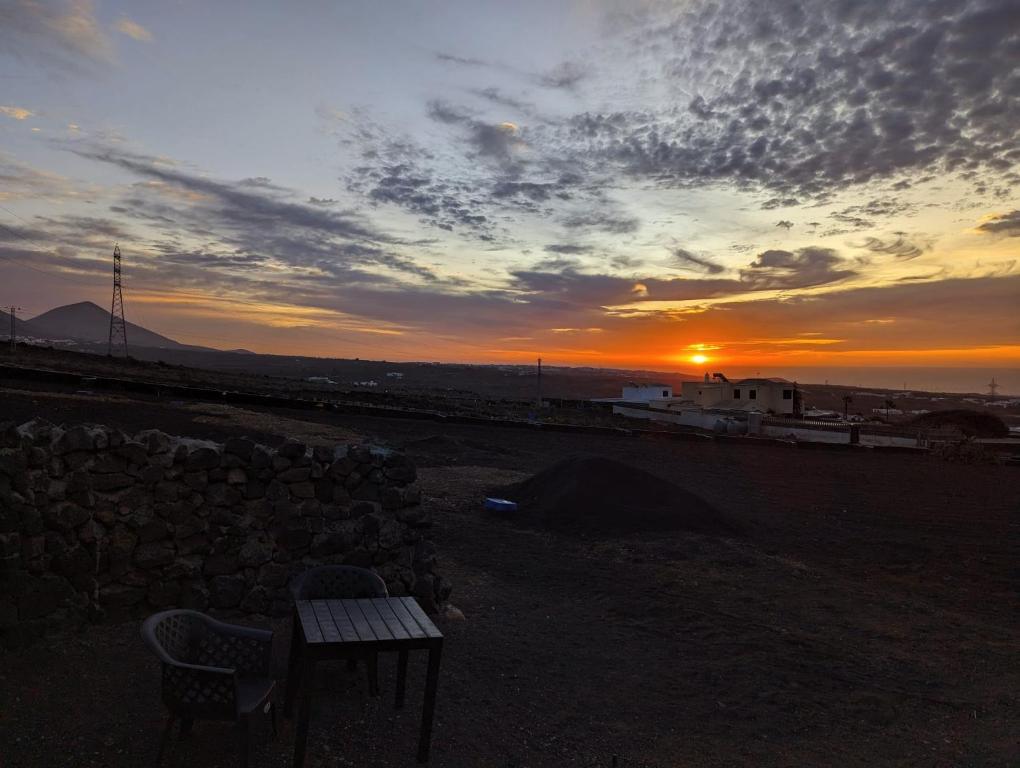As the sun sets over a desolate stretch of land, an image unfolds capturing the essence of a remote and potentially undeveloped area. The sparse landscape suggests a possible farm or work site, characterized by an absence of substantial buildings. However, a single, distant structure on the right hints at agricultural activity, perhaps for processing crops or grain, indicated by an outcropping used for loading materials. In the foreground, on the left side, a small table accompanied by two plastic and metal chairs sits next to a large stack of firewood, evoking a sense of rural living where morning coffees might be enjoyed amidst the rustic setting. The terrain is flat and treeless, with only bushes and tumbleweeds dotting the expanse. A prominent pile of dirt lies in the middle of the scene, and there appears to be a trailer, indicative of someone residing on-site. Overhead, clouds drift across the sky, adding to the dusky ambiance as the day transitions into night, casting a somber mood over this seemingly impoverished area.